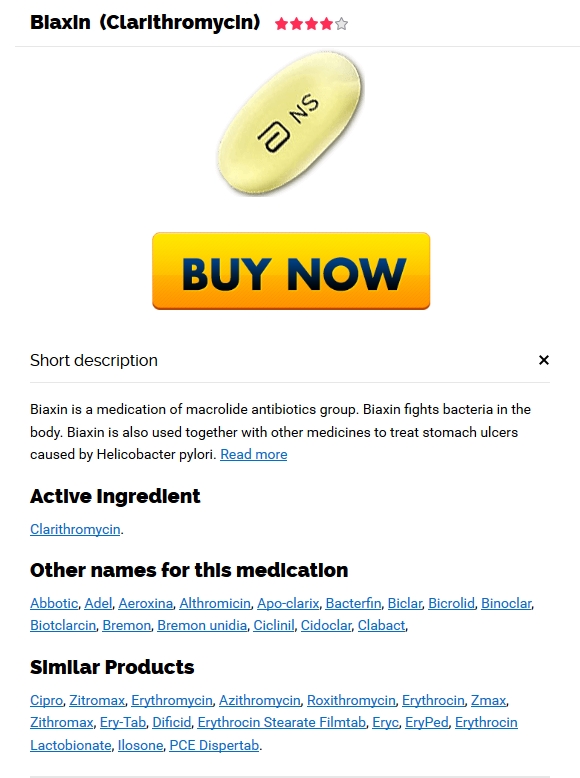**Caption:**

This image showcases a detailed webpage for a prescription drug named Blaxin, which is also known by its active ingredient, Clarithromycin. The webpage has a clear title with "Blaxin" prominently displayed at the top. Directly underneath, the alternative name "Clarithromycin" is provided. The drug is represented with a four-star rating.

The image depicts the pill itself, which is oval and yellow, marked with an "S" and a large, upside-down "E". A prominent yellow button labeled "Buy Now" invites users to make a purchase.

A short description elaborates that Blaxin belongs to the macrolide antibiotics group and is effective against bacteria in the body. It is also prescribed in combination with other medications to treat stomach ulcers caused by Helicobacter pylori.

The caption lists additional names for Clarithromycin, including Abotic, Adele, Eroxima, Athrowiass, Apocler, Clarix, Baxctofin, Byclar, Bycrowlid, Notclar, Bioclar, Claire soon, and Selenia Seto Clar. Additionally, the related products section mentions similar antibiotics such as Cipro, Zithromax, Ethramycin, Eroxmycin, E-Mycin, Z-Max, and many more.